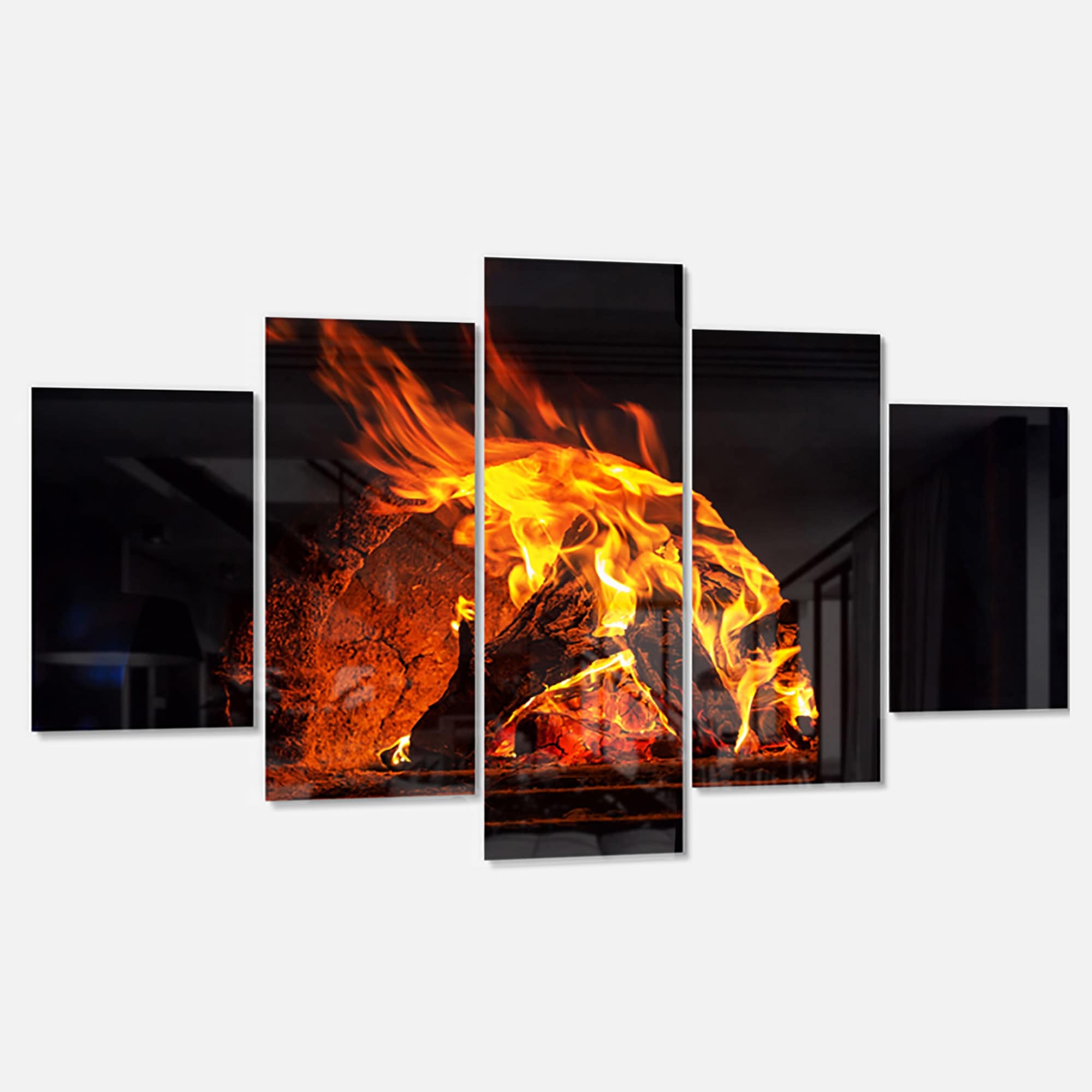The image shows a digital fireplace composed of five glass panes arranged in an ascending and descending order by size. Starting from the left, the sizes of the panes increase towards the center and then decrease symmetrically towards the right. The three central panes prominently display a vivid scene of burning logs, with bright yellow and orange flames enveloping red-hot wood. The two outermost panes, one on each side, show partial reflections of the burning material and some gray and black railings in the background. The entire setup is framed with low, unobtrusive borders against a predominantly gray backdrop, giving a modern and minimalist aesthetic to the digital fireplace on the wall.